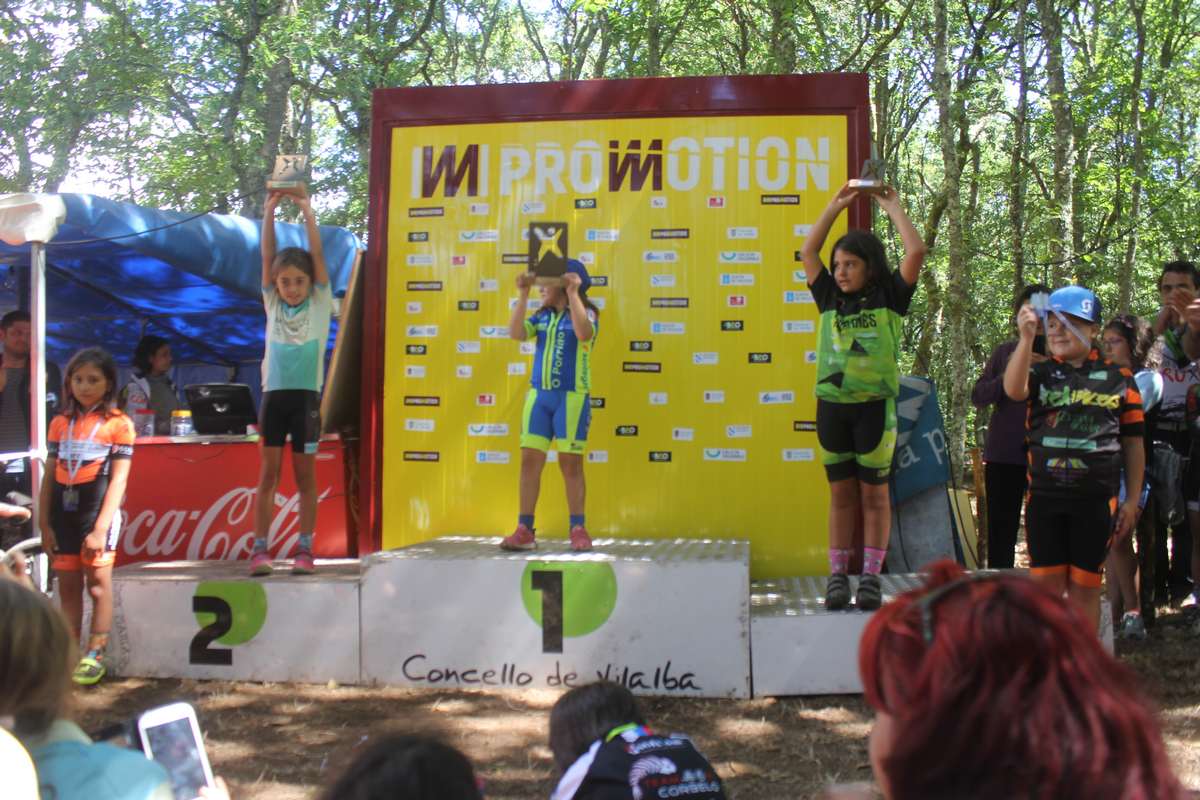In this vibrant outdoor scene, a group of young children proudly stands on an award podium, celebrating their achievements in what appears to be a race or contest. The podium is set against a backdrop of lush trees, with spectators gathered around to watch the ceremony. 

The podium has three levels: the tallest in the center marked "1," flanked by shorter platforms labeled "2" and "3." A large banner reading "Pro Motion" in white and brown letters against a yellow background hangs behind the podium, adorned with smaller patches likely representing sponsors.

The first-place winner, Consuelo de Villalba, stands tall on the center podium, holding her trophy high above her head. She is dressed in a blue and yellow athletic outfit. To her left, the second-place winner, a young girl in a blue shirt and black shorts, also raises her award high. The third-place winner, positioned on the right, sports a black and green jersey with matching shorts, accessorized with pink socks and black sneakers, and lifts her trophy proudly.

Beside the podium, children holding medals are lined up, adding to the celebratory atmosphere. In the foreground and around the area, people are milling about, enjoying the event, while a snack stand is visible to the left. The ground in front of the podium is bare dirt, contrasting with the vivid greenery of the surrounding forest.